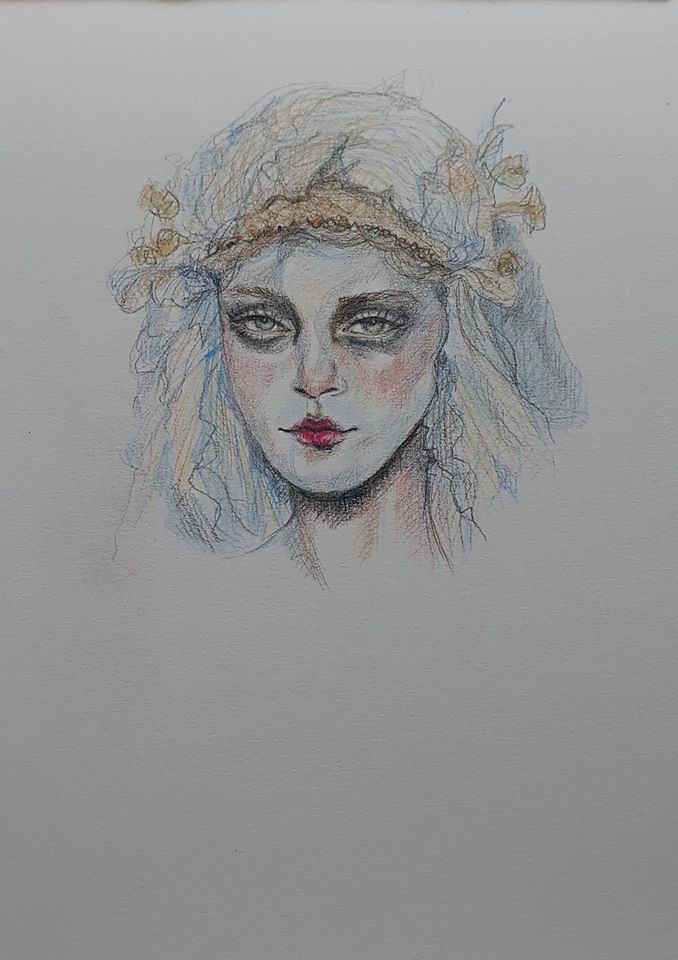The image features a detailed color drawing of a woman with long, multicolored hair resembling spaghetti, which transitions in hue and shading. The drawing appears to be created using a mix of colored pencils and standard pencils on a plain white sheet of paper. She has a crown of yellow flowers, possibly daisies or carnations, adorning her forehead and interspersed in her hair. Her face is very expressive, with pale skin and steel gray, forward-staring eyes, framed by dark, heavily shaded makeup. Her lips are vividly colored in red. The artwork includes varying red and black shading on her cheeks and neck, although some areas show cross-shading errors where colors blend into unintended sections. Despite these imperfections, the image captures a striking and intensely focused expression.